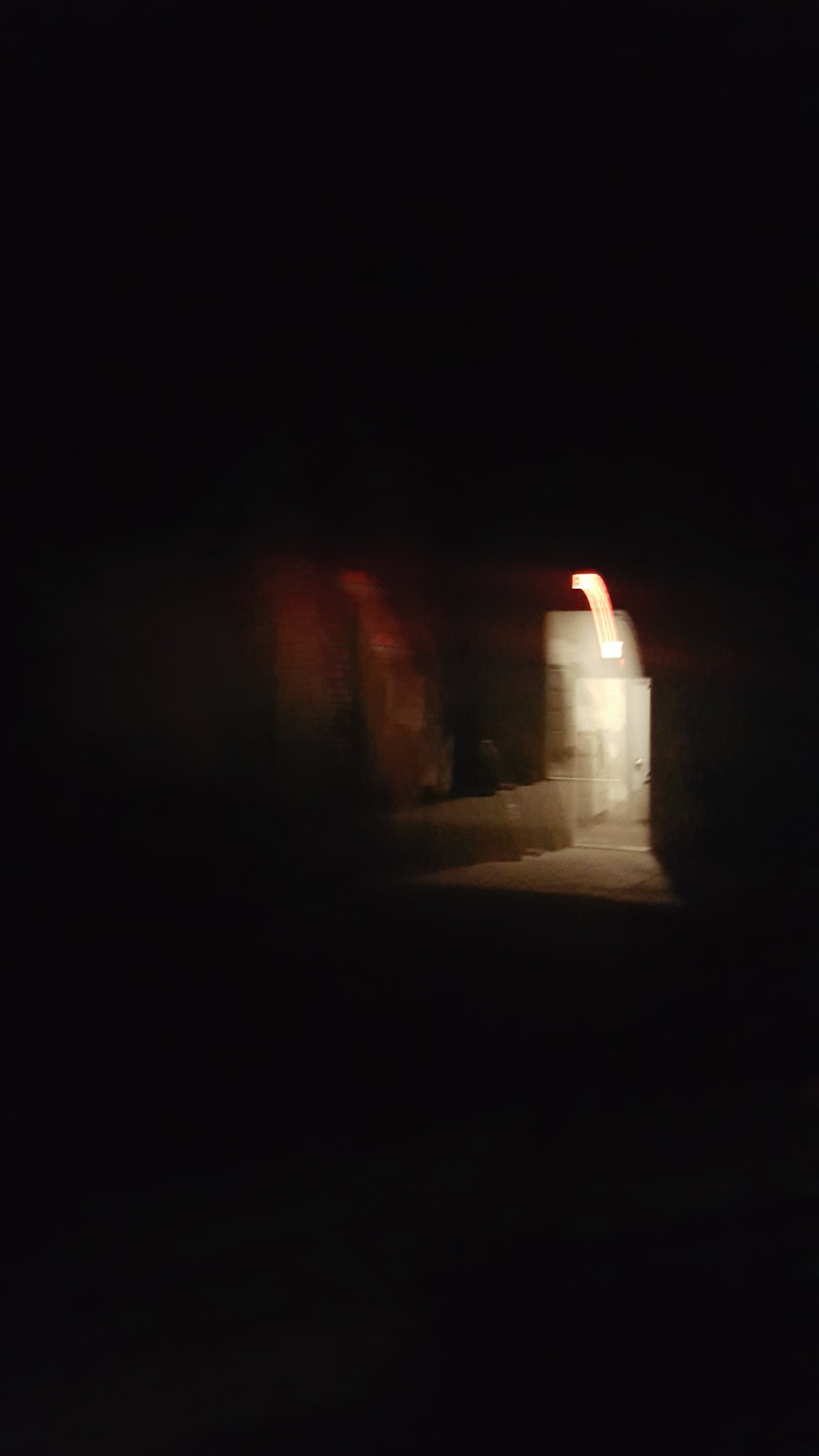A very dark and blurry photograph captures the interior of an indistinct location. The predominant feature is an illuminated doorway at the center, starkly contrasting against the surrounding blackness. The doorway, possibly marked by an exit sign above, emits a bright light that appears streaked, hinting that the photo was taken in motion. This illuminating glow spills out, faintly lighting up a section of the floor with no discernible details visible.